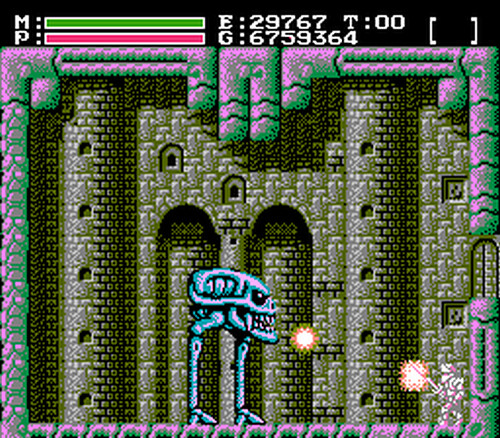The image captures a pixel art screen from an old-school 8-bit video game, reminiscent of a scene from Super Ghouls 'n Ghosts. The screen is nearly a perfect square, with a black letterbox occupying the top 10-15%. This area displays two bars: a green one labeled 'M' and a red one labeled 'P', likely representing various game metrics such as health or power. Additionally, there are numerical indicators prefixed by 'E:', 'G:', and 'T:', whose exact meanings are unclear, alongside empty brackets in the upper right perhaps meant for items or weapons.

The main visual focuses on a dynamic encounter set against a castle backdrop marked by green and pink highlights. A knight-like character, positioned at the bottom right wielding a sword, confronts a menacing skull-faced creature. This creature, resembling an alien skull with elongated bone-like legs and some fangs, hovers menacingly while emitting fireballs towards the knight. The skull creature has a malicious grin and an extended cranium. Scattered light beams add to the dynamic tension of the scene, suggesting an intense, chaotic battle.